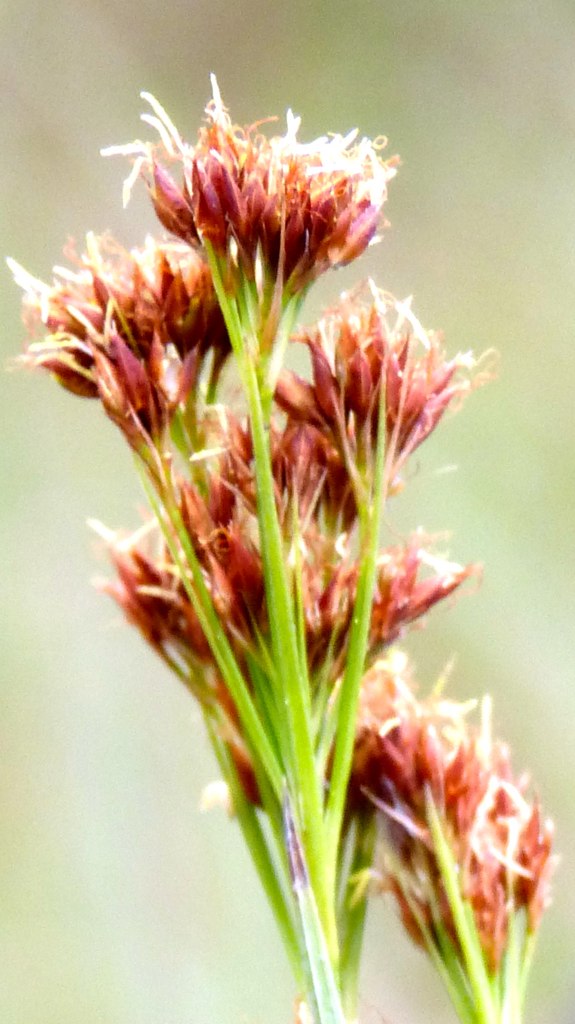This image captures a vibrant cluster of freshly bloomed flowers. Each flower exhibits a unique gradient of colors, starting with a striking purple-brownish hue at the petals, transitioning to a delicate light yellow at the very tips. The flowers are grouped together in dense clusters atop slender, vibrant green stems, adding to their lush appearance. Adjacent to this central cluster is another similar bunch, showcasing the abundance and healthiness of the blossoms. The background features a soft light green shade, further highlighting the vividness of the flowers and creating a harmonious, natural setting.